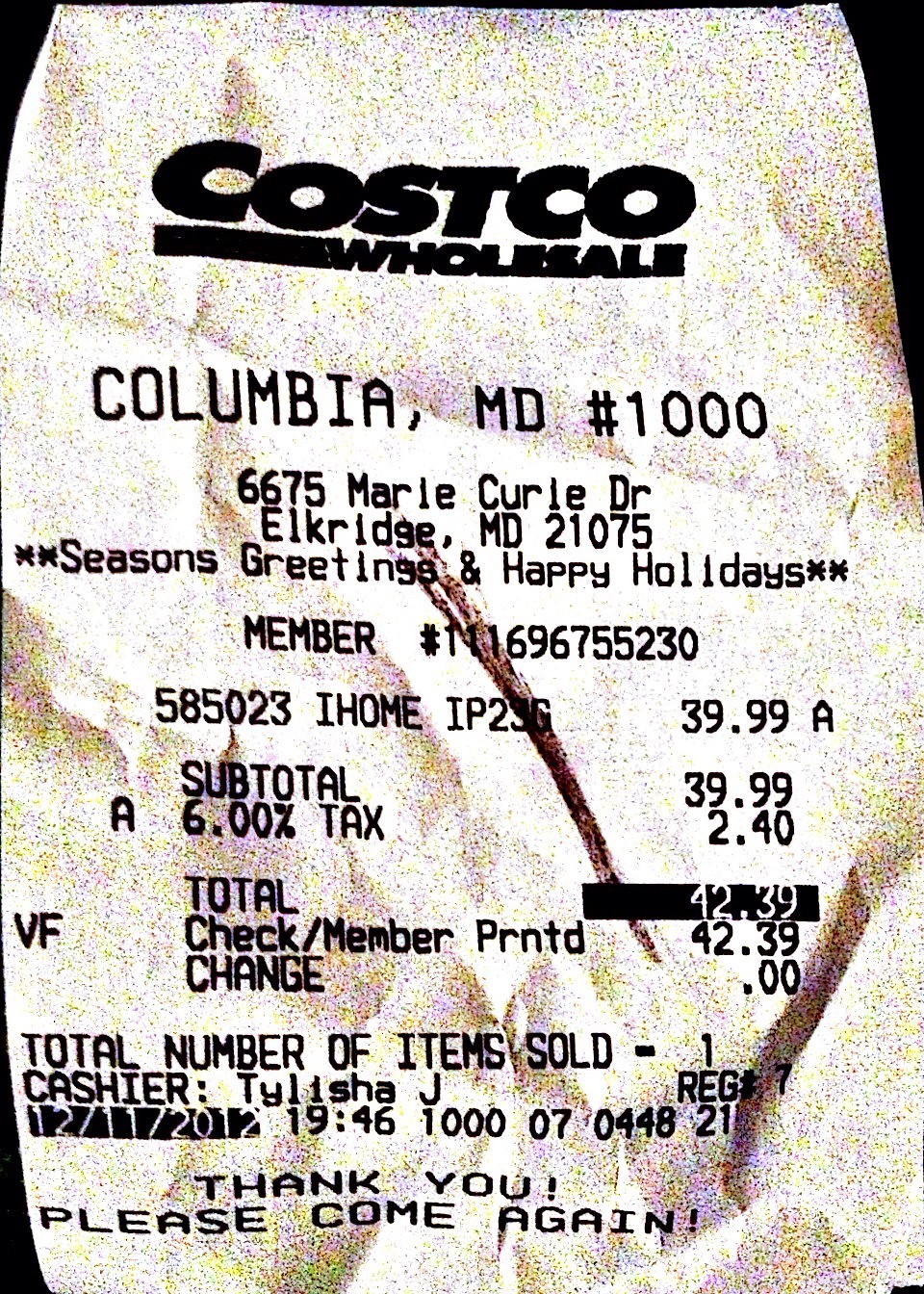A grainy, photocopy-like image features a receipt with numerous stray black marks and shading inconsistencies. The top of the receipt prominently displays the Costco logo, with the word "Costco" above and "Wholesale" below a dividing line. The backdrop behind the receipt is entirely dark. The receipt indicates the location as Costco in Columbia, Maryland, identified by store number 1000, situated at 6675 Marie Curie Drive, Elkridge, Maryland, 21075. A festive message, "Season's Greetings and Happy Holidays," is printed on the receipt. Further details include itemized purchases and the total amount. The date and time at the bottom are marked as 12-11-2012, 19:46.